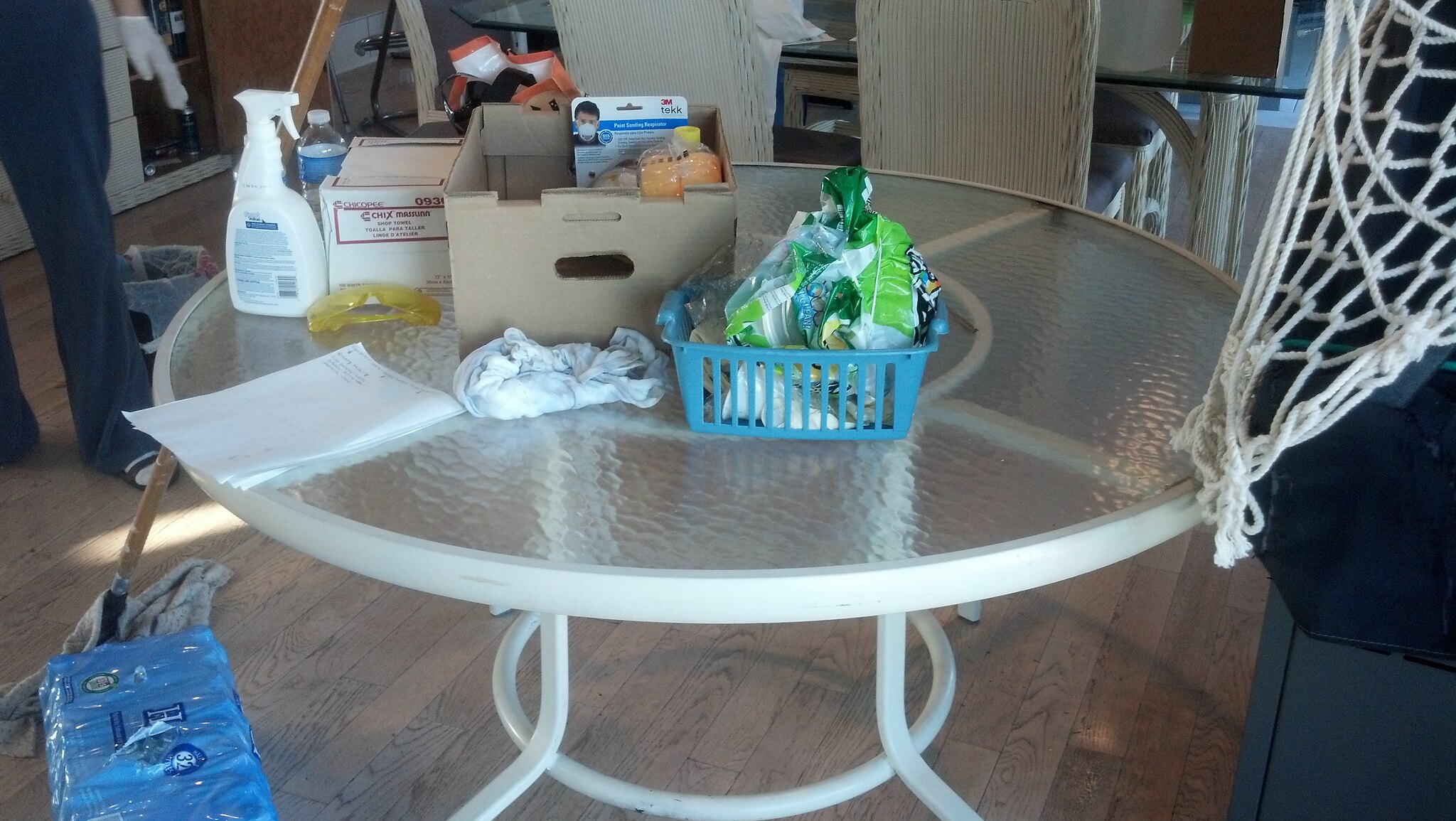This detailed photo captures a circular tempered glass table situated in what appears to be a living room or dining area. The table features a white rim and white legs that extend outward from a central circle, adding a modern touch to the space. Atop the table, there are various cleaning supplies, including spray bottles, rags, and boxed masks, indicating an ongoing cleaning session. A small blue crate, possibly used for collecting trash, is also present. On the floor beside the table lies a large pack of plastic water bottles. In the far left-hand corner, a person wearing sweatpants and latex gloves—possibly paired with socks or sandals—stands, evidently engaged in the cleaning process. To the right, a net-covered object suggests protective measures are being taken to shield it from cleaning products or debris.